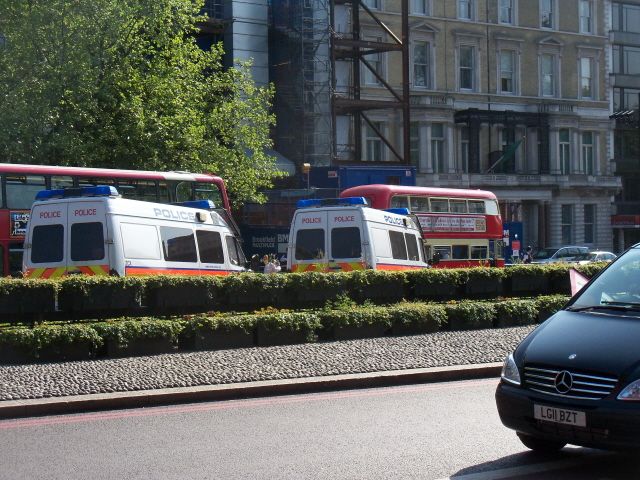The photograph captures a bustling street scene in London, featuring a dual carriageway with two lanes on each side and a central raised pavement adorned with cobblestones and small hedges. In the foreground, the nose of a black Mercedes people carrier with the registration LG11BZT is just entering the frame. Across the road, two police riot vans marked with "POLICE" in red and blue print and equipped with blue and red lights are prominently positioned. Near them, a classic red London double-decker bus, likely used for a tourist trip, is visible alongside a standard London Red bus and several other vehicles. Lining the street are old-style buildings with bay windows, typical of London’s architectural heritage. A large leafy tree rises from the pavement, adding to the picturesque scene. Additionally, far in the background, tall apartment buildings can be seen, some possibly undergoing maintenance as suggested by the scaffolding. Scattered pedestrians add life to the sidewalks of this charming, busy London street.